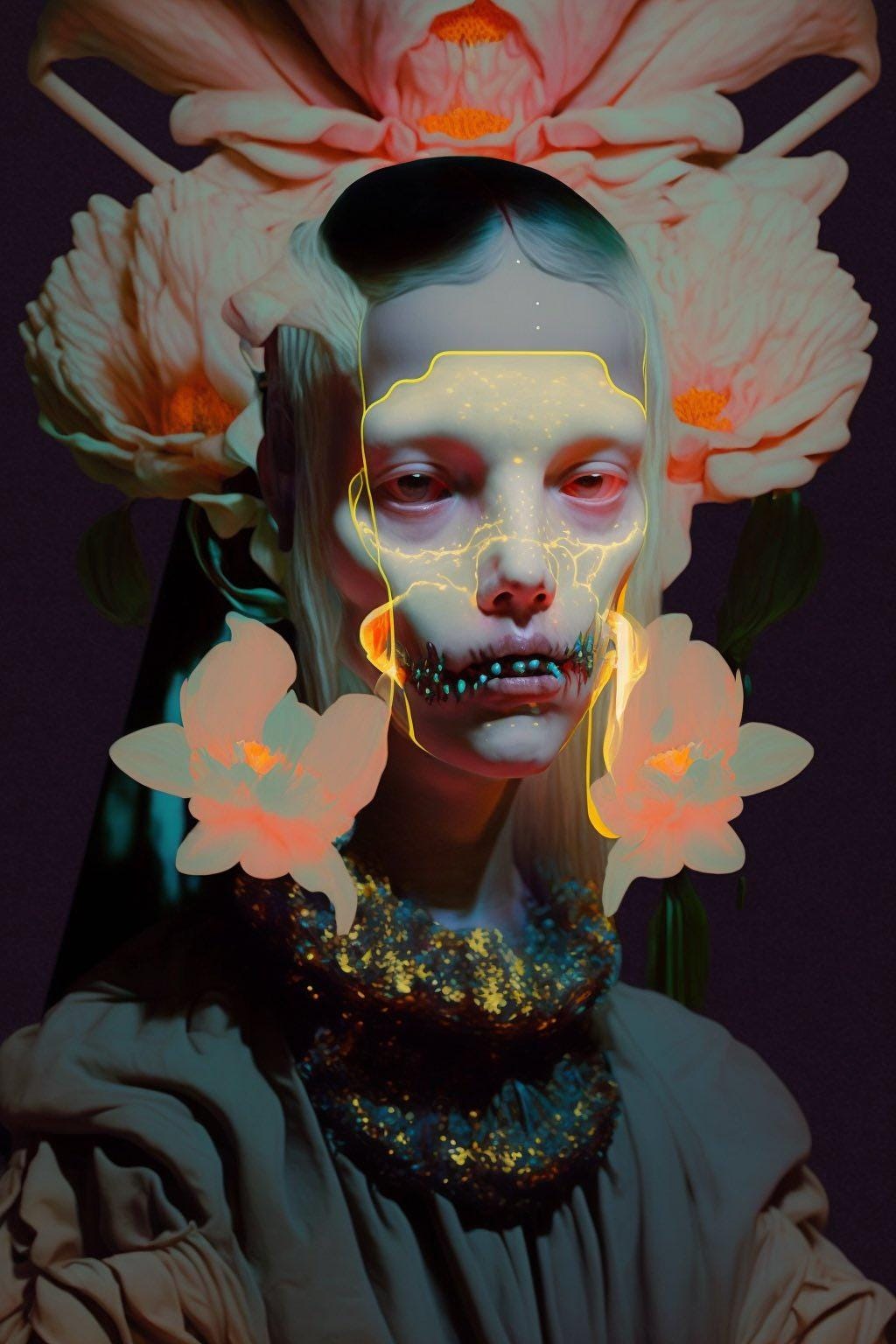The image presents a hauntingly ethereal woman in a dark, moody composition that combines photography with digital painting. Her head is crowned with vibrant pink flowers boasting bright orange centers, giving an almost surreal floral headpiece effect. Her face bears an unsettling, skeletal appearance with deep-set, almost crossed eyes and a mouth adorned with unsettling green teeth. Golden frames encircle her eyes and jaw, adding a touch of ornate surrealism. Surrounding her elongated neck are two additional flowers and wreaths, blending seamlessly with her crumpled tan blouse, which possesses a flowy, classical aesthetic reminiscent of couture fashion. The dark background is contrasted by a cool blue light that enhances the eerie, demon-like vibe. The overall ambiance is both artistic and editorial, creating a beautiful yet disturbing portrait that defies conventional beauty standards.